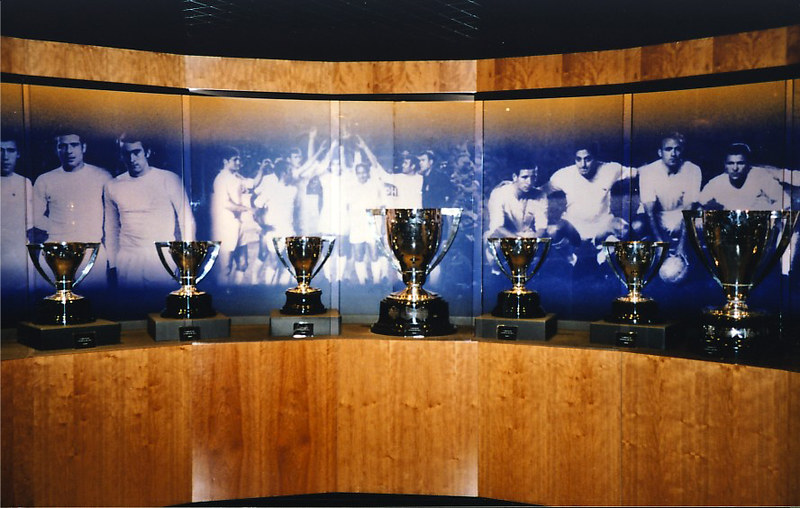This detailed photograph showcases a museum-like setting with a curved wooden wall adorned with seven gold trophy cups. The background features a mix of black and orange-brown tan paneling strips. The top part is black, with the orange-brown wood paneling forming a curved design below it. Black and white photographs with a blue tone of sportsmen dressed in white uniforms reminiscent of the 1950s to 1970s adorn the wall. These vintage images, depicting teams with their arms around each other and squatting in front of a ball that appears more like a rugby ball, enhance the nostalgic atmosphere. There is a shelf in front of these photographs holding the seven gold trophies. The arrangement includes five medium-sized trophies and two significantly larger ones, with the larger ones positioned at the center and right end of the shelf.